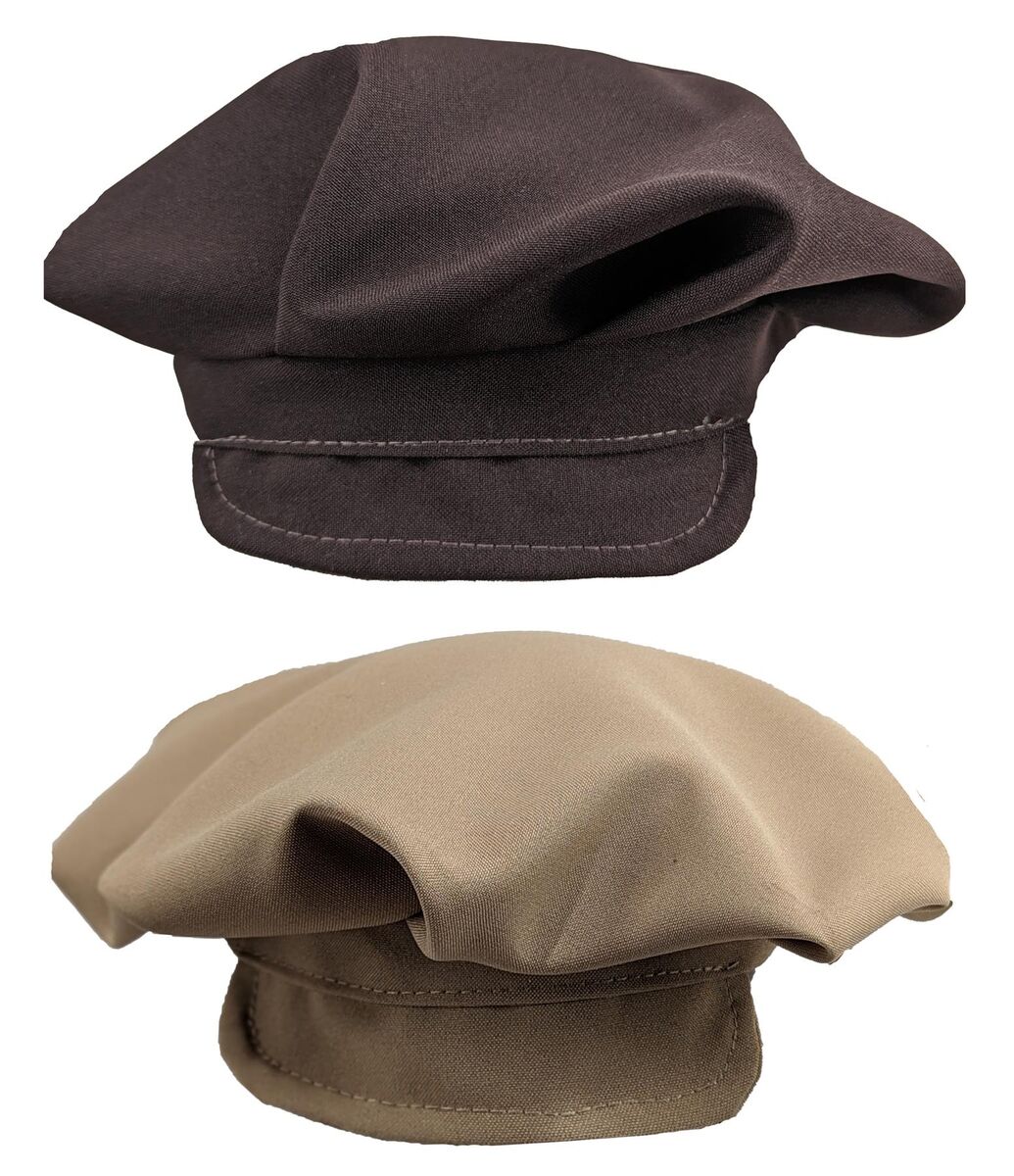The image features two hats with a distinctive mushroom-like shape, characterized by a rounded, puffy top and a narrower lower brim. Both hats share a similar soldier or European style, reminiscent of a French beret or paperboy cap. The top hat is a dark greenish-purple or dark grayish-purple, appearing almost brown in certain lighting. It has visible white stitching and is slightly folded over at the top part. Below it, the second hat is a beige or light tan color, mirroring the first hat's design with a downward-pointing brim and similar folding. Both hats are aligned vertically on a plain white background, with a light source accentuating the fabric texture and minor shadows under the brims.